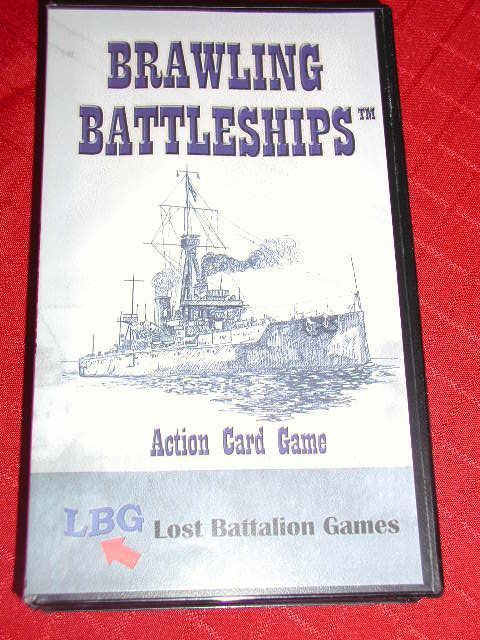The image depicts a square object placed against a red background with a woven diamond pattern. It appears to be a game box for "Brawling Battleships™," featuring predominantly white and gray colors with purple lettering. The main title, "Brawling Battleships™," is written in an old-fashioned, large font. Below the title is a line drawing of a battleship on the water, complete with smoke plumes, tall masts, and a small flag. Underneath the illustration, it says "Action Card Game." At the very bottom, a dark blue-gray strip displays the letters "LBG" with an arrow pointing towards them, next to the words "Lost Battalion Games." The entire box is showcased in a plastic protector resembling a clamshell VHS case.